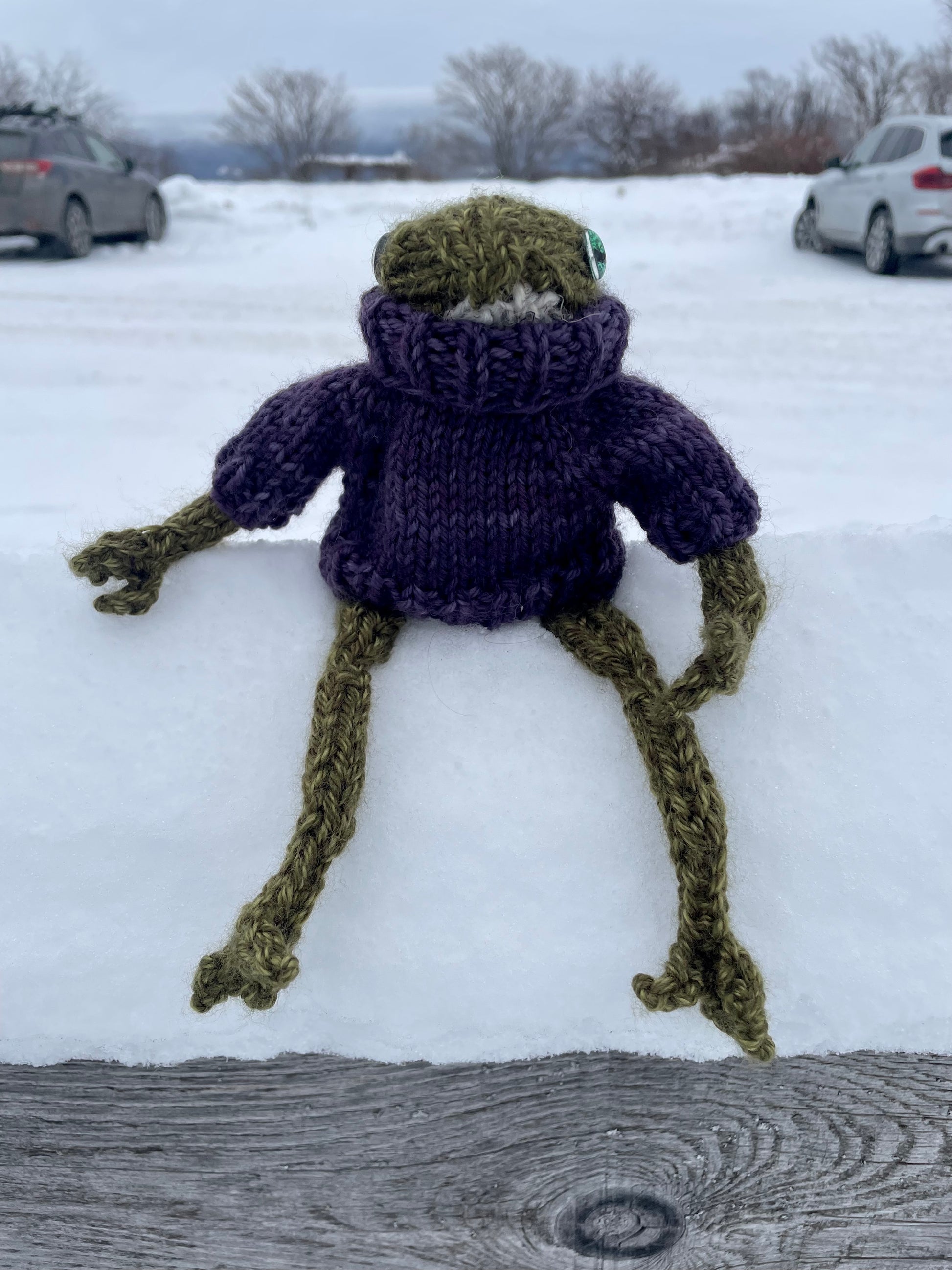The image is a detailed color photograph with a portrait orientation, showcasing a handcrafted crocheted frog. The frog, primarily olive green with green hair, is adorned with a high-collared purple (or possibly dark blue) turtleneck sweater that nearly obscures its face. Its googly eyes peek out from the sweater's high collar, giving it a whimsical appearance. The frog's four long, thin limbs are made of green yarn, with its legs hanging over the edge of a short snow-covered wall, nearly touching the ground. The wall itself has a section where the wood is exposed and grey, featuring some lines and a circular wooden ring. Beyond the wall, the background reveals a snowy area with two parked cars, leafless trees, and a grey sky. The composition portrays a detailed, realistic scene that captures the handcrafted nature of the frog toy amidst a wintery setting.